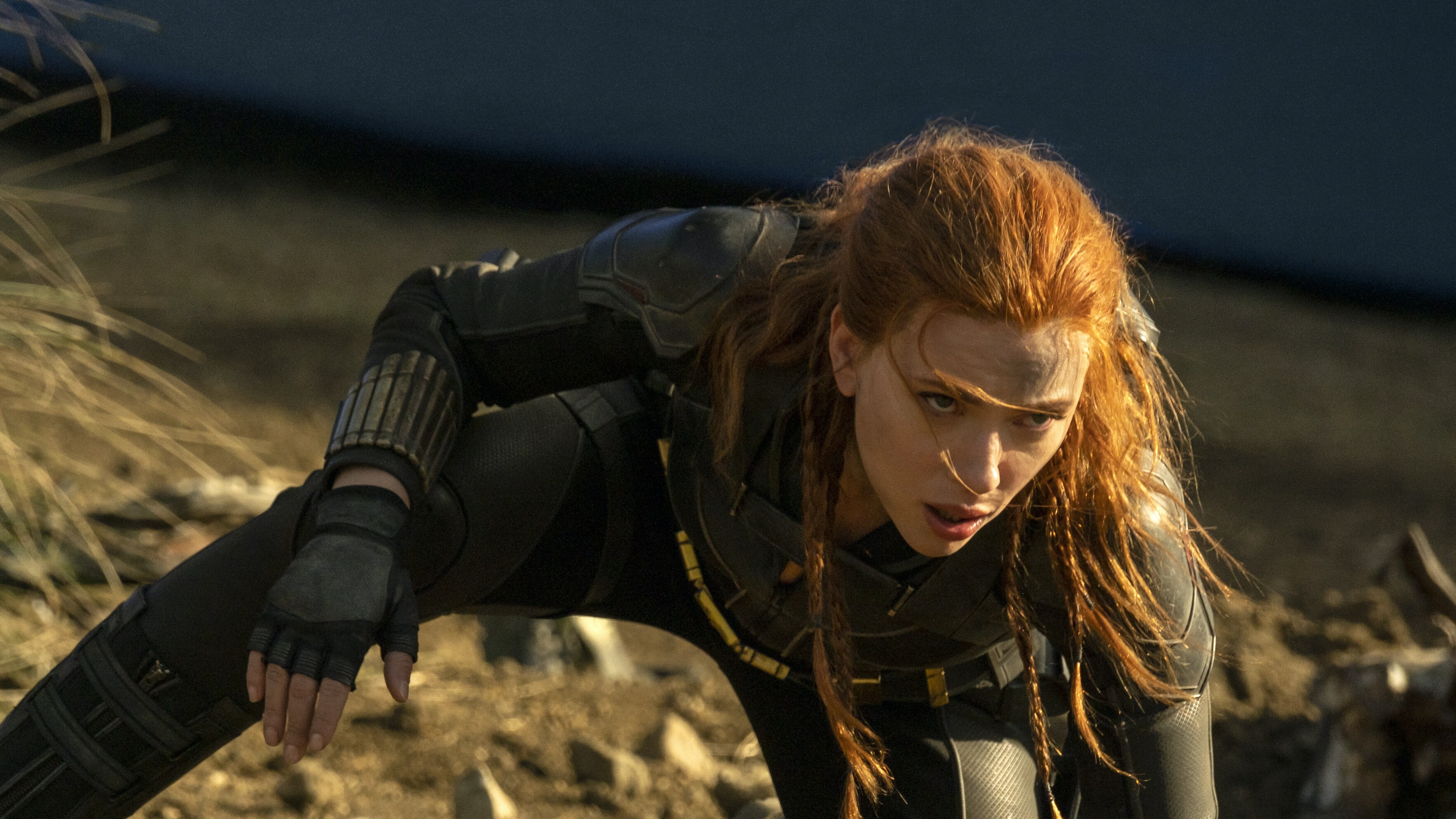In this action-packed scene from what appears to be a television show or movie, a woman is captured in a crouched, ready-to-run stance that exudes intense focus and determination. She is dressed in a superhero-like outfit, reminiscent of Marvel characters, which includes dark leather pants and a long-sleeved, shoulder-padded shirt. Her ensemble also features fingerless gloves on her right hand. Her red hair, partially braided, falls against her face, which is marked by smudges of dirt, indicating the gritty environment she is in. The background reveals a blurred, rocky, and grassy field with hints of a blue lake in the distance, adding to the rugged, outdoors setting of the shot. The woman, who is Caucasian, has a competitive, almost fierce expression, underscoring the dramatic intensity of the moment.